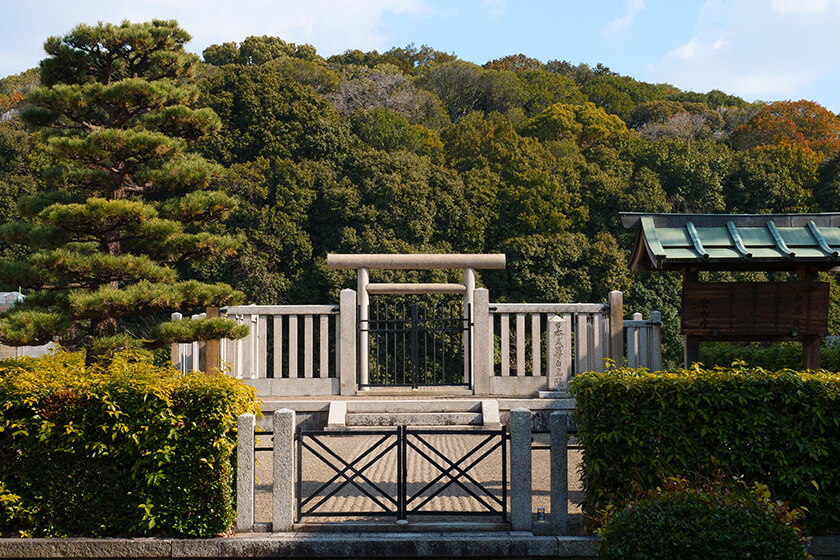This photograph captures a serene scene with distinct Asian architectural influences. In the foreground, there are two lush, but moderately unkempt, deciduous hedges flanking a black metal gate. The gate, split into two swinging doors, features a prominent X-shaped design and is supported by sturdy concrete pillars. Beyond this gate lies a courtyard that appears to be made of sand or gravel, meticulously raked, suggesting it might be part of a Zen garden.

To the right of this entrance is an eye-catching structure: a wooden sign with Japanese characters, sheltered by a curved green roof, indicative of traditional East Asian design. This structure has water pipes and a metal bar extending across its peaked roof. Immediately next to it is a pergola. On the left side of the gate, there is a large evergreen tree, sculpted to resemble a bonsai, adding to the tranquil ambiance.

The scene extends to another black metal gate at the far end of the courtyard, again supported by concrete pillars and topped with a horizontal concrete bar. The fence continues with evenly spaced vertical pillars. In the background, lush, green, forest-like trees cover a hilly landscape, reaching up to a blue sky patterned with a few feathery clouds. The overall composition and intricate details strongly suggest a traditional Japanese garden or temple setting, evoking a sense of peace and meticulous design.